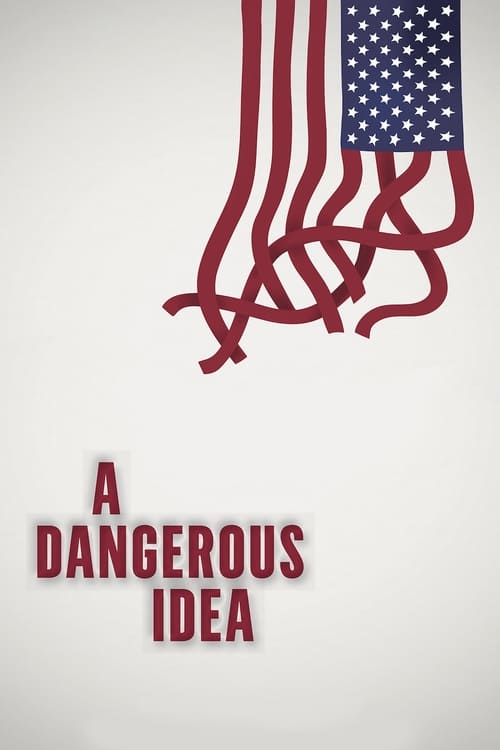The image depicts an American flag rotated 90 degrees and positioned in the upper right corner against a vertically aligned light grayish-white background. The blue section with white stars remains intact, while the red stripes cascade downward like twisted ribbons, giving the appearance of unraveling and falling apart. In the lower left corner, bold red text with a shadow effect spells out "A dangerous idea" across three lines. The overall composition is stark and minimalistic, emphasizing the distressed flag and the provocative message, suggesting the cover of a book or a political poster.